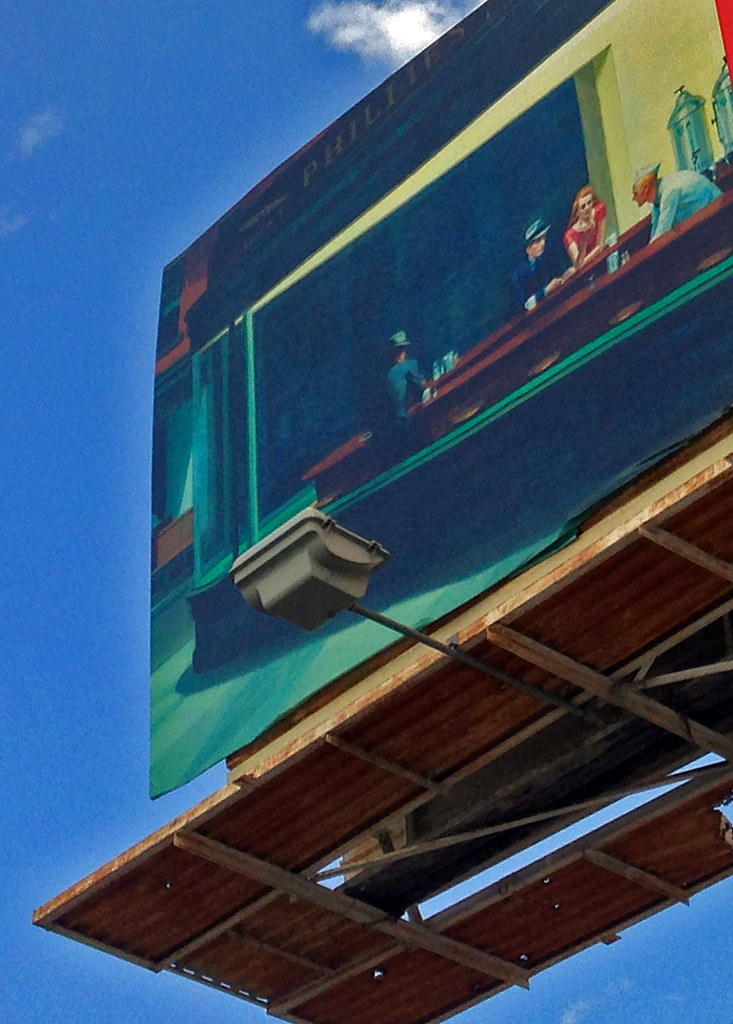In this image, a billboard set against a light medium blue sky features a scene from a bar. The billboard's graphic shows a man possibly at work, dressed in a blue jumpsuit and matching blue cap, sitting by himself. In the background, the bartender is bent over, seemingly in the process of grabbing or placing an item. In the foreground, a man and a woman are standing across the bar from the bartender, leaning forward as if engaged in conversation. The woman is wearing a striking red dress, while the man is dressed in a sharp blue suit, with both of their arms resting on the bar. Scattered white clouds add a touch of calmness to the sky behind the billboard.